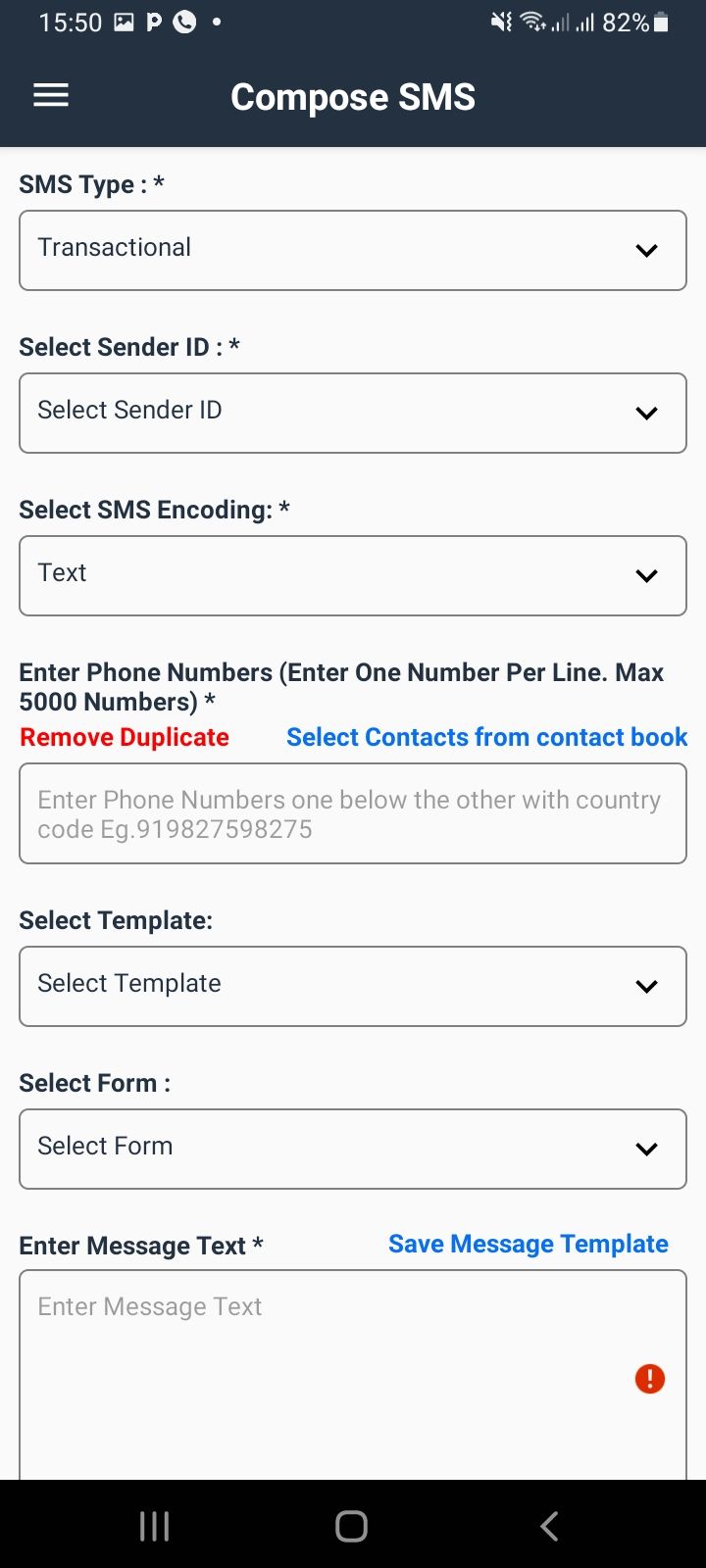This screenshot, captured from a mobile phone, displays a user interface for composing an SMS. At the top left corner, the current time is shown in military format as 15:50, accompanied by several icons. On the top right corner, additional icons are visible: vibration mode, Wi-Fi status, signal strength, an 82% battery indicator, and battery percentage icon.

Below these indicators, the main interface for SMS composition is presented. The SMS type is set to "Transactional". The option to select a "Sender ID" is available but currently not inputted. The SMS encoding is set to "Text". Users can input phone numbers with a maximum limit of 5,000 numbers, one per line. There are options to remove duplicates or select contacts from the contact book.

Further down, the interface provides an option to select a template and a form, both of which currently have no selections made. The message text area is empty, awaiting user input. Finally, options to "Save Message Template" is provided, but no text has been entered.

At the bottom of the screen, the navigation bar includes settings, home, and back buttons.